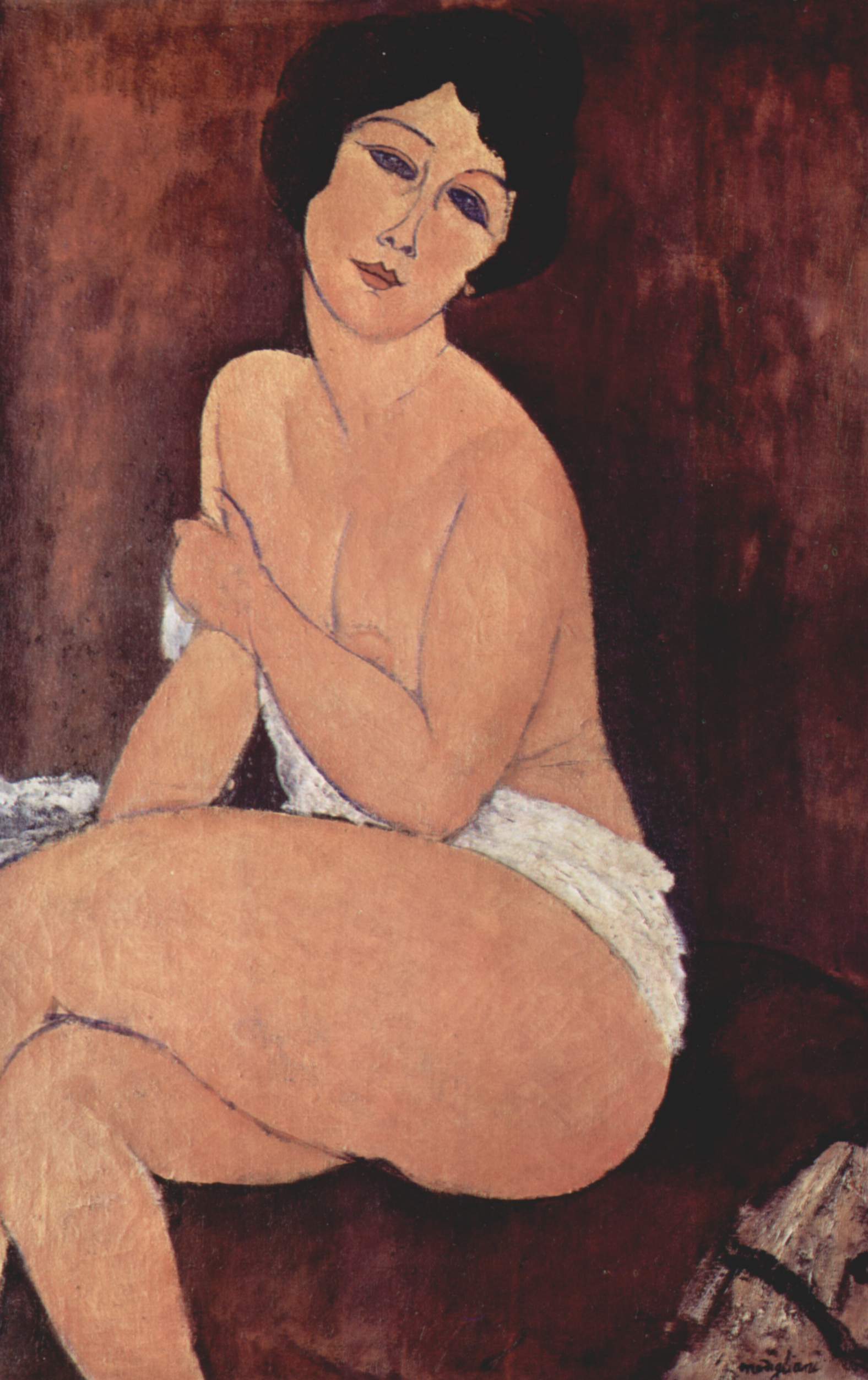The artwork is a painting of a woman with short black hair and striking blue eyes, exuding a seductive aura as she gazes directly at the viewer. The woman is mostly unclothed, with her left arm strategically positioned to cover her right breast while her left breast is partially exposed, showing a bit of areola. She wears a deep red lipstick, enhancing the sensuality of her pose. Her left leg is bent over her right, which is positioned closer to the viewer. A white towel or dress drapes over her left thigh and hip, extending to cover around her right elbow. The background is a gradient of dark to light red, with an oddly detailed stone featuring a black tie visible on one side. The painting's style appears somewhat amateurish, with exaggerated features and uneven proportions, evoking an old flapper girl aesthetic. The crude depiction and distinctively large eyes impart an almost alien quality to her appearance. The woman is seated on what seems to be a red couch, blending into the similarly colored background.